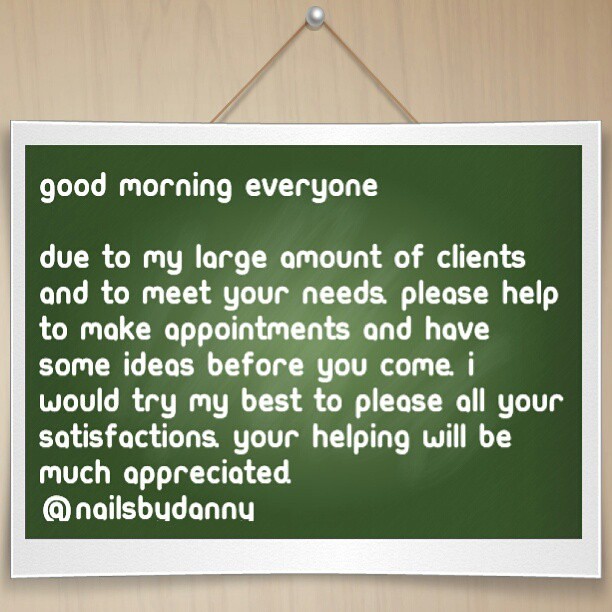This is a descriptive sign for "Nails by Danny," seemingly aimed at clients of a nail salon. The sign features a green background with white text and a silver-white border, resembling a school chalkboard. It reads, "Good morning everyone. Due to my large amount of clients and to meet your needs, please help to make appointments and have some ideas before you come. I will try my best to please all your satisfactions. Your helping will be much appreciated." The sign is rectangular, hangs from a wall via a darker brown string attached to a pearly white knob, and is set against a lighter wood background. Danny appears to be asking clients to schedule appointments to better accommodate their needs, suggesting his services are quite in demand. The text structure indicates that English may not be the native language of the writer.